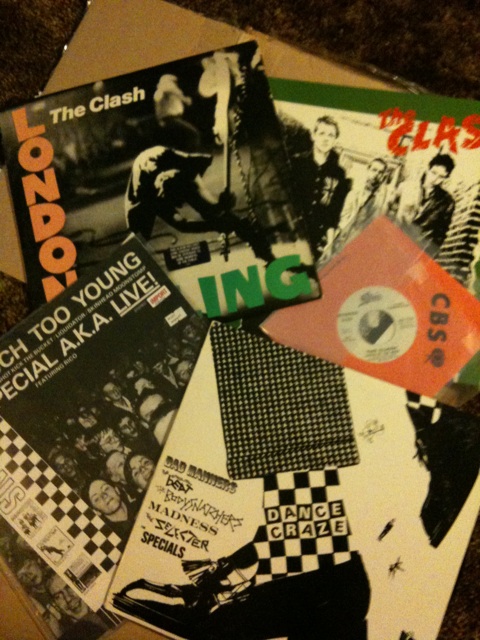The image depicts a fan-like arrangement of various records and record albums on a black countertop. Dominating the top left is the iconic "London Calling" album by The Clash, featuring the album's title in a vertically placed London text on the left and "The Clash" in white to the right, partially obscured by overlapping records. Adjacent to it, slightly overlapping, is an album with a crowd of concertgoers under a title ending in "ING" in green, visible at the left-hand edge, with the words "Too Young, Something Live" partially legible in white across the top. Covering this, at an angle from bottom left to top right, is an album depicting a person's lower leg, ankle, and black shoe; it prominently displays "Dance Craze" on the ankle, with some partially obscured black text to the left. Above this, a smaller record in an orange case with visible black text and a central white label peeks out. Completing the arrangement is another album by The Clash at the top, showing the band in a stylized red drawing.